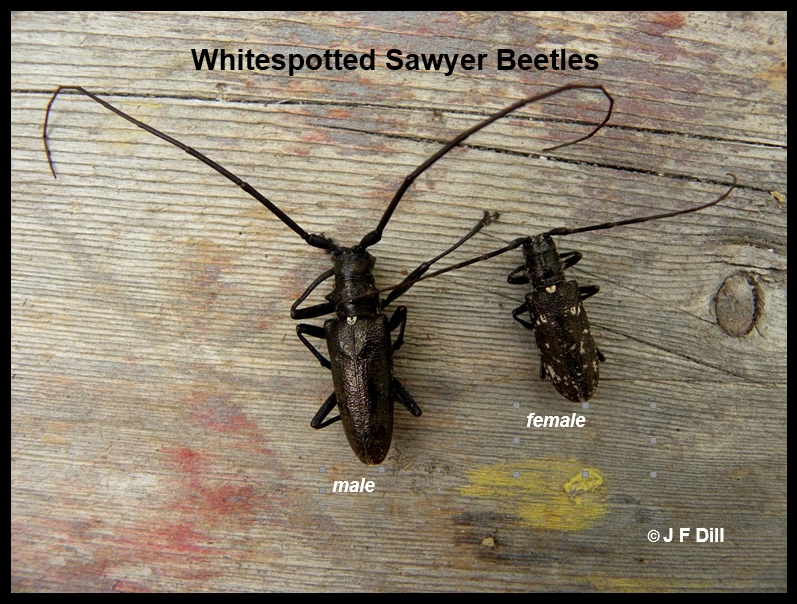The image features a detailed photograph of two White-Spotted Sawyer Beetles, labeled as such in black lettering at the top. Both beetles are set against a weathered, splotchy wooden surface resembling that of a park table or deck, exhibiting red and yellow residue marks. Central to the composition, the male beetle is situated on the left and identified by the white text "male." This beetle, characterized by a large oval body, six legs, extremely long antennae, and a distinct heart-shaped white spot on the back of its neck, is predominantly dark brown to black. To its right, the smaller female beetle is labeled "female" in white text. Like the male, she has six legs and long, though slightly shorter, antennae, with numerous lighter spots accentuating her dark brown to black coloration, including a similar heart-shaped marking. The photo is credited to J.F. Dill, as noted in the bottom right-hand corner.